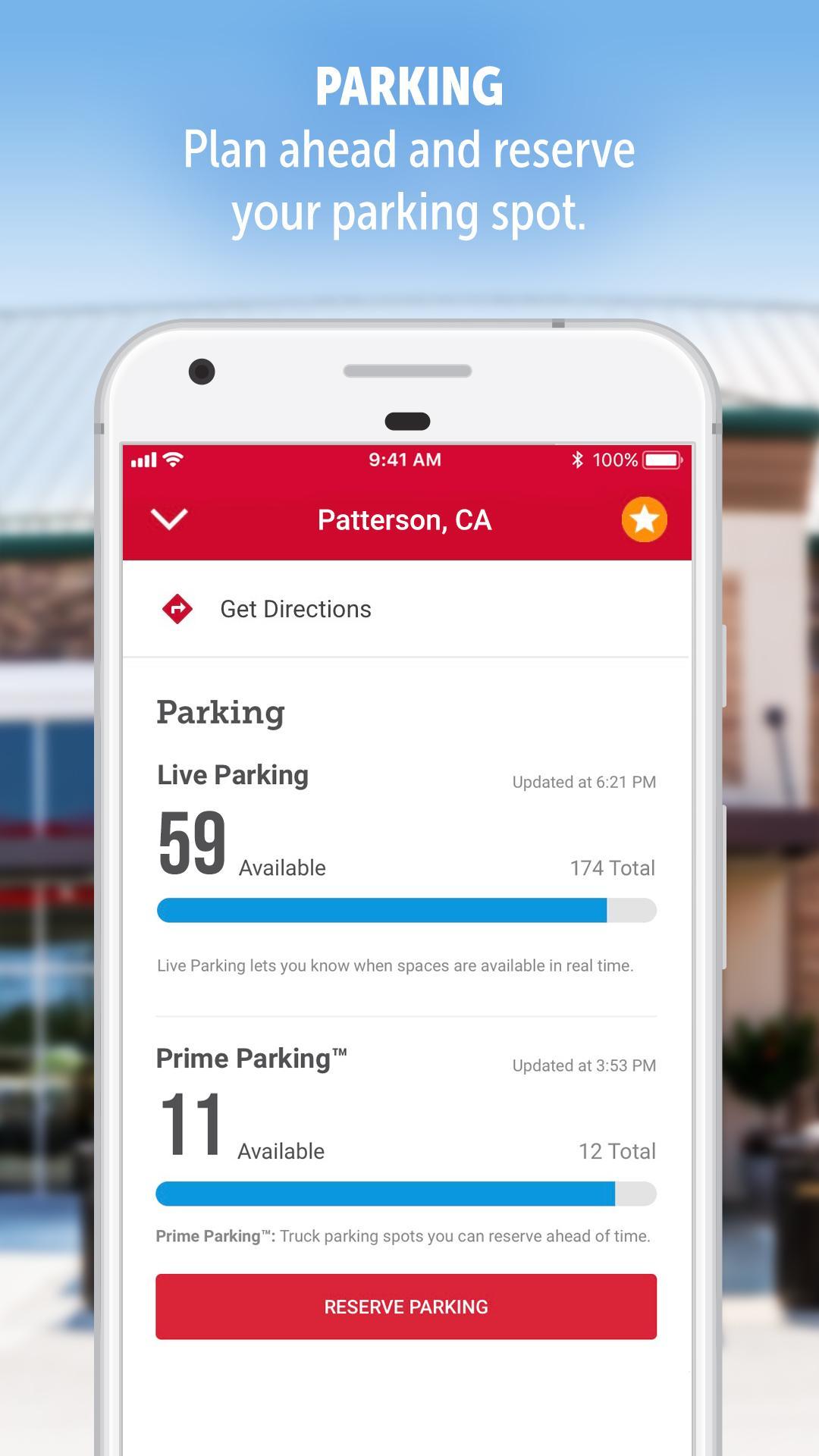The image presents a front view of a smartphone with a white frame. The phone's screen is on, displaying a user interface overlaid with text and graphics. The top of the screen features a bold red bar with the text "Paterson, California" prominently displayed. Just beneath this red bar, the screen shows an option labeled "Get Directions."

The main portion of the screen has a white background with the word "Parking" written on the left side. Directly below this is the heading "Live Parking" followed by the information "59 available," accompanied by a blue status bar indicating parking availability.

The background of the overall image features a clear blue sky with the text "Parking Plan Ahead and Reserve Your Parking Spots" written in white across it. A building, serving as the backdrop for the main image, is visible below the sky-text, providing context and environment to the primary subject of the image.